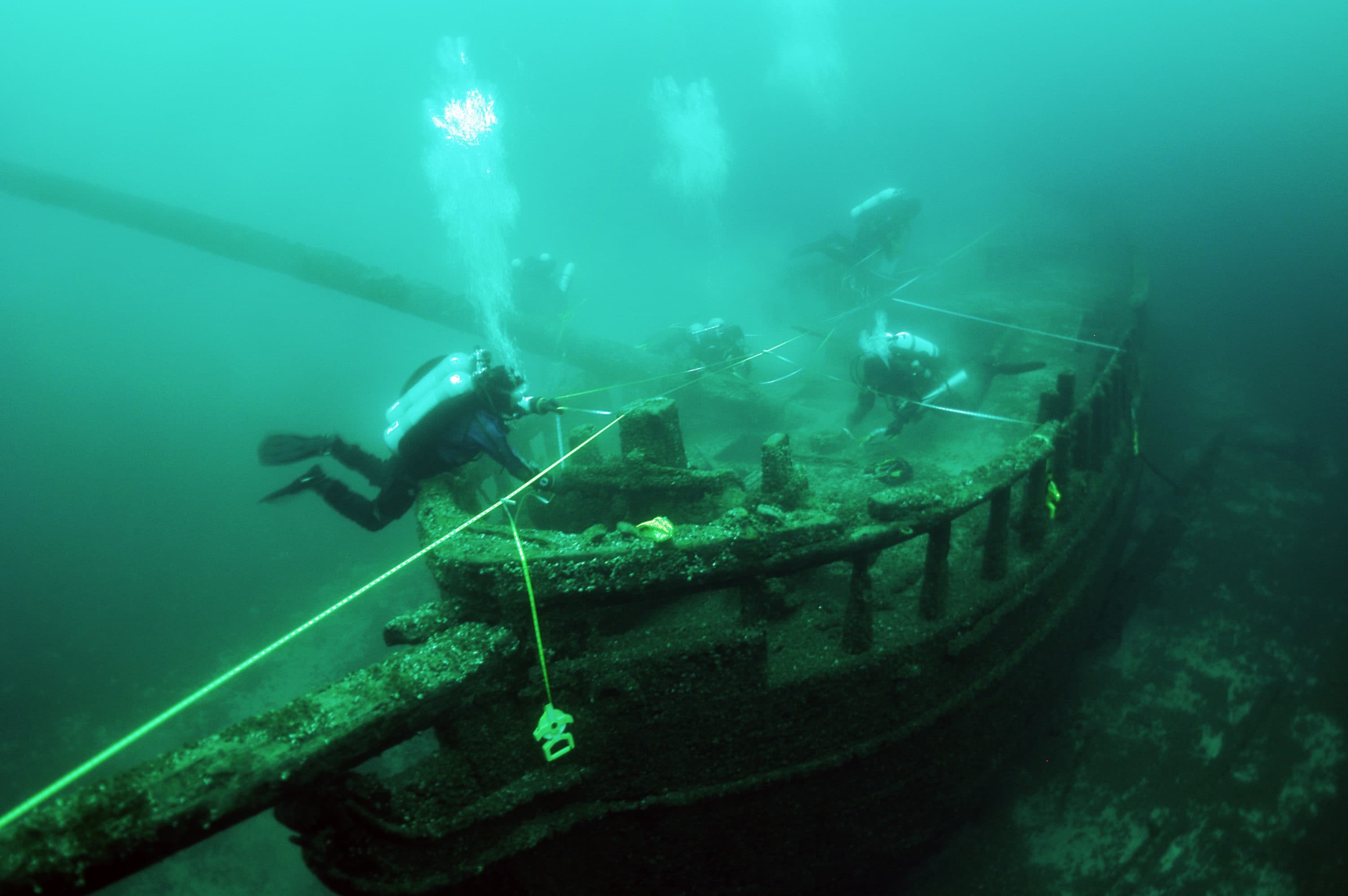In this underwater photograph, a group of five to six scuba divers in black suits—with light blue oxygen tanks and black fins—are meticulously exploring and attaching yellow ropes around an ancient wooden shipwreck at the murky bottom of the ocean. The weathered, brown ship is covered in barnacles, moss, seashells, and anemones, indicating it has been submerged for a significant period. The hull suggests it could have housed about ten sailors, and appears to resemble a 15th-century caravel. Part of the mast is broken and tips towards the seafloor, poking out from the middle of the vessel. The surrounding seabed features patches of sand and ocean floor, enhancing the dramatic discovery scene. Overall, the divers' bubbles ascend as they work, highlighting the intriguing, historic nature of their find amidst the sunken relic.